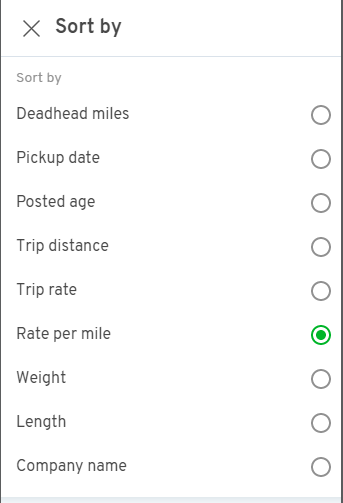A screenshot of an application interface is displayed. On the left side, there is a black "X" button, presumably for closing the window. The background of the interface is white, with "Sort By" written in grey at the top. Along the right-hand side, several clickable options are presented, each contained in a bubble. These options include "Deadhead Miles," "Pick Up Dates," "Posted Age," "Trip Distance," "Trip Rate," "Rate Per Mile," "Weight," "Length," and "Company Name." When a bubble option is highlighted, it turns green. In this screenshot, the "Rate Per Mile" option is specifically highlighted and circled in green, indicating it is the selected sorting criterion. A grey line is present at the bottom of the application interface, adding a subtle boundary to the design elements.